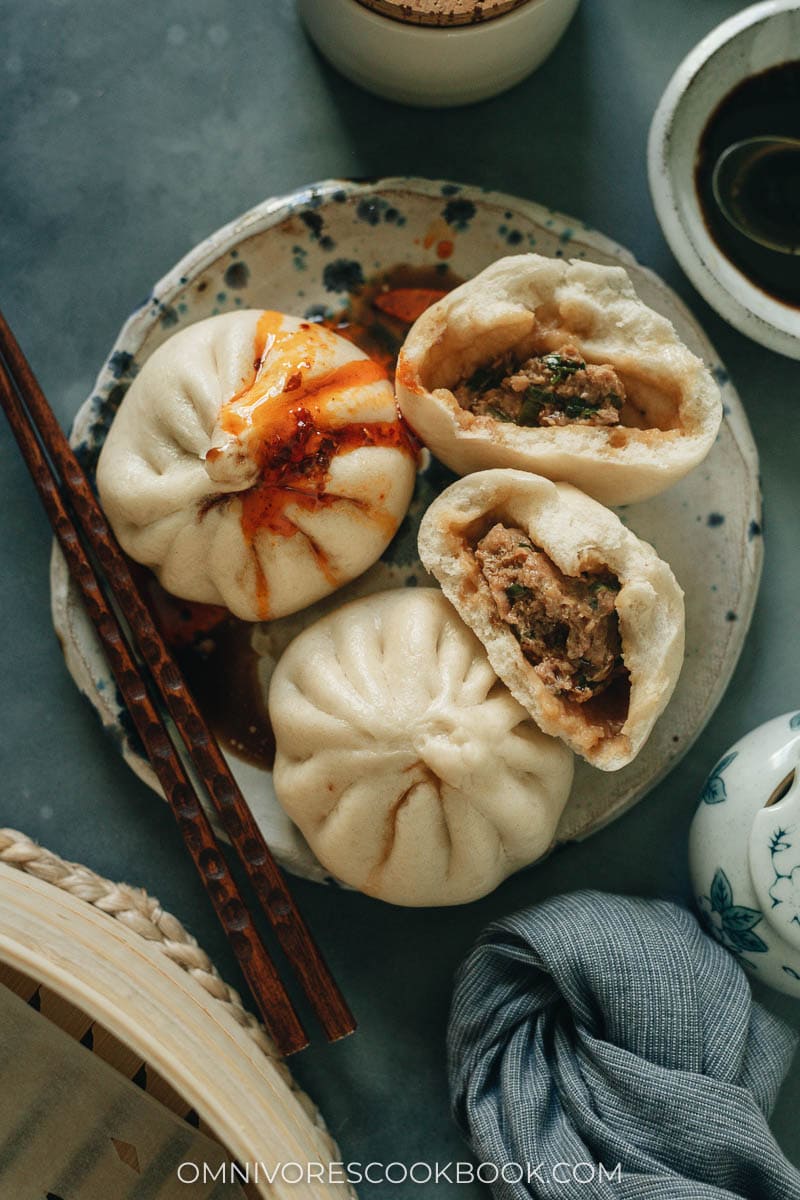The photograph showcases a top-down view of a small, white plate with green and orange speckles, positioned in the center of the frame. On the plate are four steamed buns, also known as Asian buns or pork buns. Two of the buns, located at the center left, are whole with a distinctive pointed and twisted top, resembling an onion or pumpkin shape. The other two buns, situated to the right, have been cut in half, revealing a savory pork filling of a brownish hue. One of the whole buns is topped with a red chili sauce or glaze. Resting across the bottom left of the plate is a pair of dark brown wooden chopsticks. The plate is set on a blue-gray tabletop, adorned with additional items including a partially visible dark blue cloth at the bottom right, some bowls, and a container near the top right that might contain soy sauce or a similar dark liquid. Also visible is a cropped basket at the bottom left. The image includes the text "omnivorescookbook.com" in small white font at the bottom.